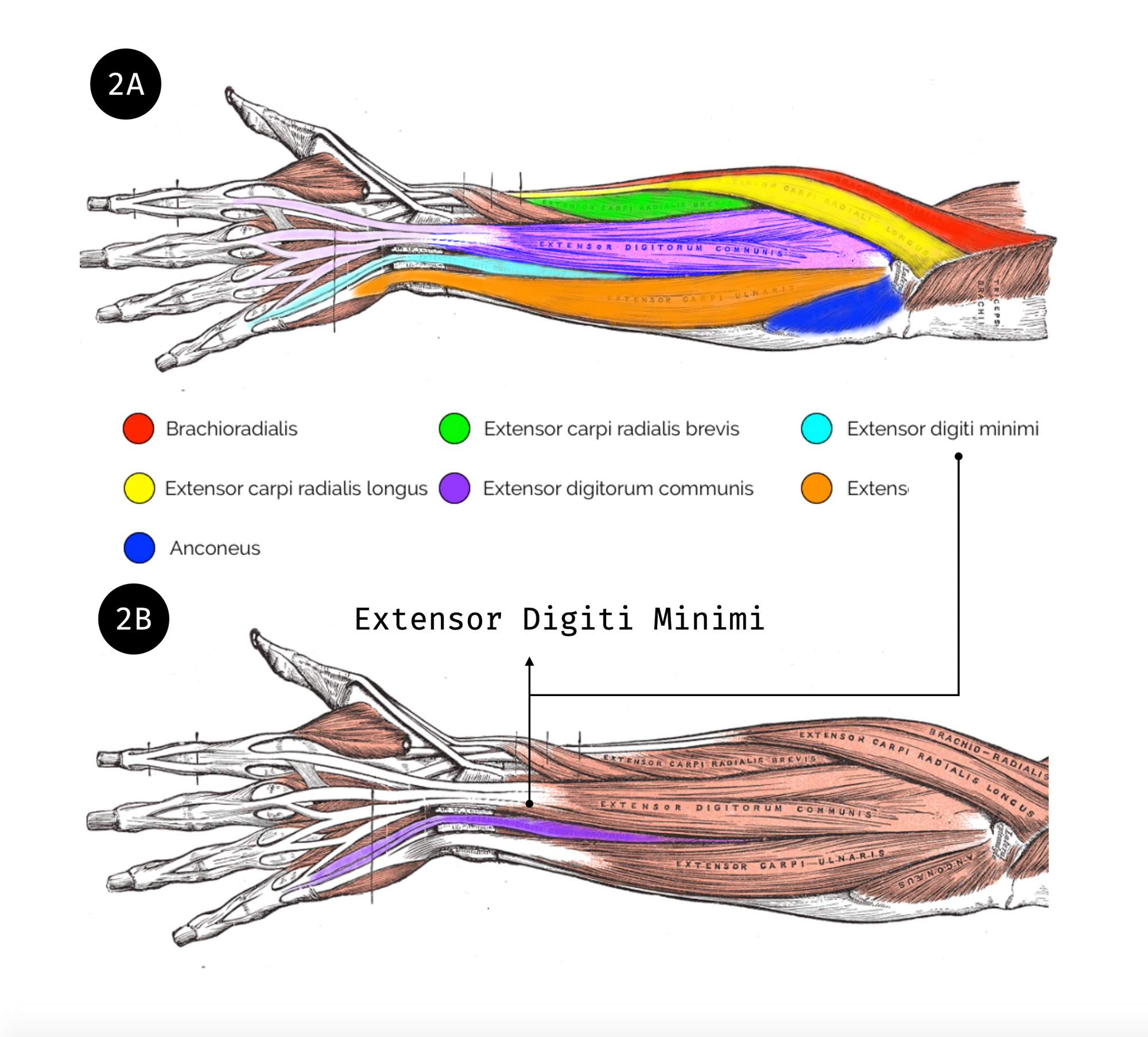The image depicts a detailed, hand-drawn schematic of the muscles of the forearm, divided into two sections labeled 2A at the top and 2B at the bottom. Both diagrams illustrate forearms extending from just below the bicep to the hand, oriented to the left side of the image. The top diagram (2A) is vibrantly colored, showcasing seven distinct muscles and tendons, each labeled and color-coded for clarity: the brachioradialis in red, extensor carpi radialis longus in yellow, anconeus in blue, extensor carpi radialis brevis in green, extensor digitorum communis in violet, extensor digiti minimi in light blue, and an unspecified muscle in orange. At the center of the image, a key correlates these colors with their respective muscle names. 

In contrast, the bottom diagram (2B) focuses on the extensor digiti minimi, highlighting it in red with a corresponding label and arrow, while the rest of the muscles remain depicted in more muted colors, primarily purple. The detailed and clear illustration helps in understanding the anatomical positioning and differentiation of the forearm muscles, with each muscle meticulously labeled for educational purposes.